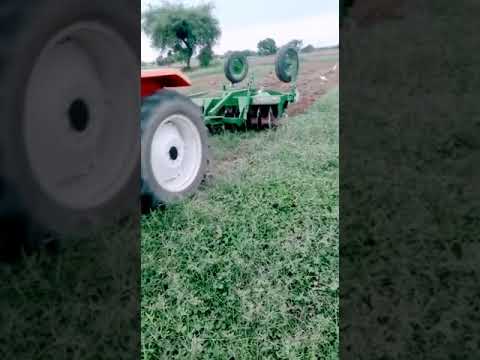The image is a vertical cell phone style shot showcasing a farming scene. Dominating the scene is the large rear tire of a reddish-orange tractor, partially visible on the left side of the image. The tractor is towing a green disc or mulching device with metal plows and multiple discs, which is actively cultivating the soil, likely in preparation for planting. The land being worked on is a flat, expansive field, partly covered with green grassy plants and transitioning to brown dirt where it has been plowed. In the background, the sky is a mix of bright white and blue, dotted with clouds, and a line of trees marks the horizon. The overall impression is of early springtime activity, with no snow and mild weather. The image itself is framed by zoomed-in and faded borders of the same scene, providing a stylish vignette effect.